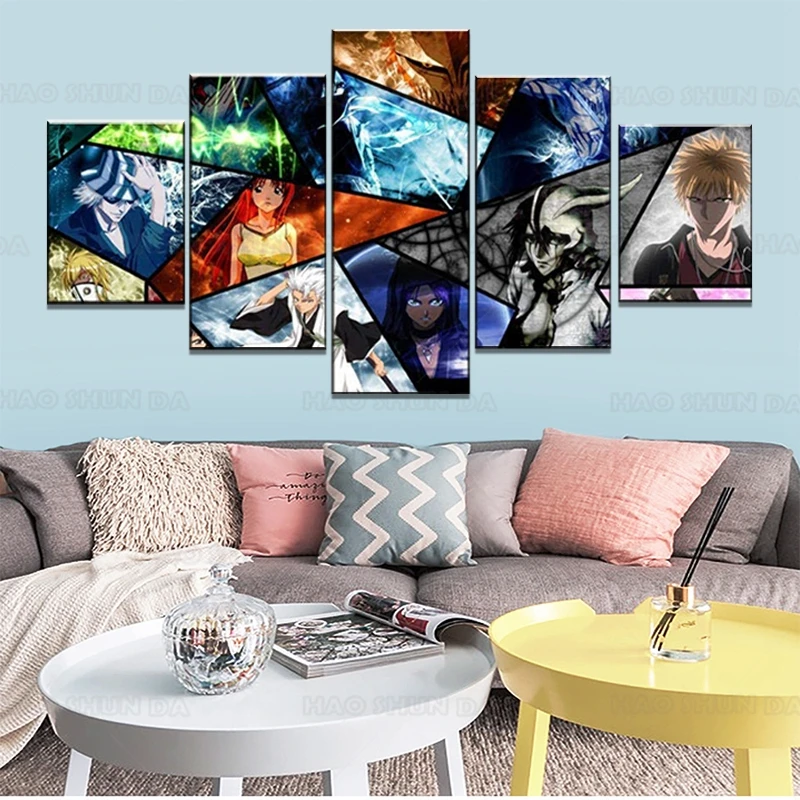This photograph captures a stylish living room featuring an array of colorful, anime-themed wall art. The wall behind the couch is painted a light blue and displays five distinct, vertically-rectangular pieces of artwork. Each piece showcases different anime characters, rendered in vivid colors such as red, blue, green, black and white, and purple. The art pieces are arranged in a horizontal diamond pattern, resembling shards of glass pieced together, giving a dynamic and cohesive look.

Below the artwork is a comfortable, brown couch adorned with various throw pillows in shades of pink, teal chevron, mint, salmon, gray, and a shaggy beige. An off-white blanket is casually draped over one side of the couch. On the floor in front of the couch lies a brown rug.

The living room also features two modern, circular coffee tables—one white and one yellow. The white table holds an open magazine next to a glass jar, possibly used for candy or potpourri, while the yellow table showcases an oil diffuser. A subtle watermark on the image reads "Haosheng DA," crediting the photographer. This inviting scene blends cozy living space with vibrant, artistic elements, highlighting the anime-themed decor.